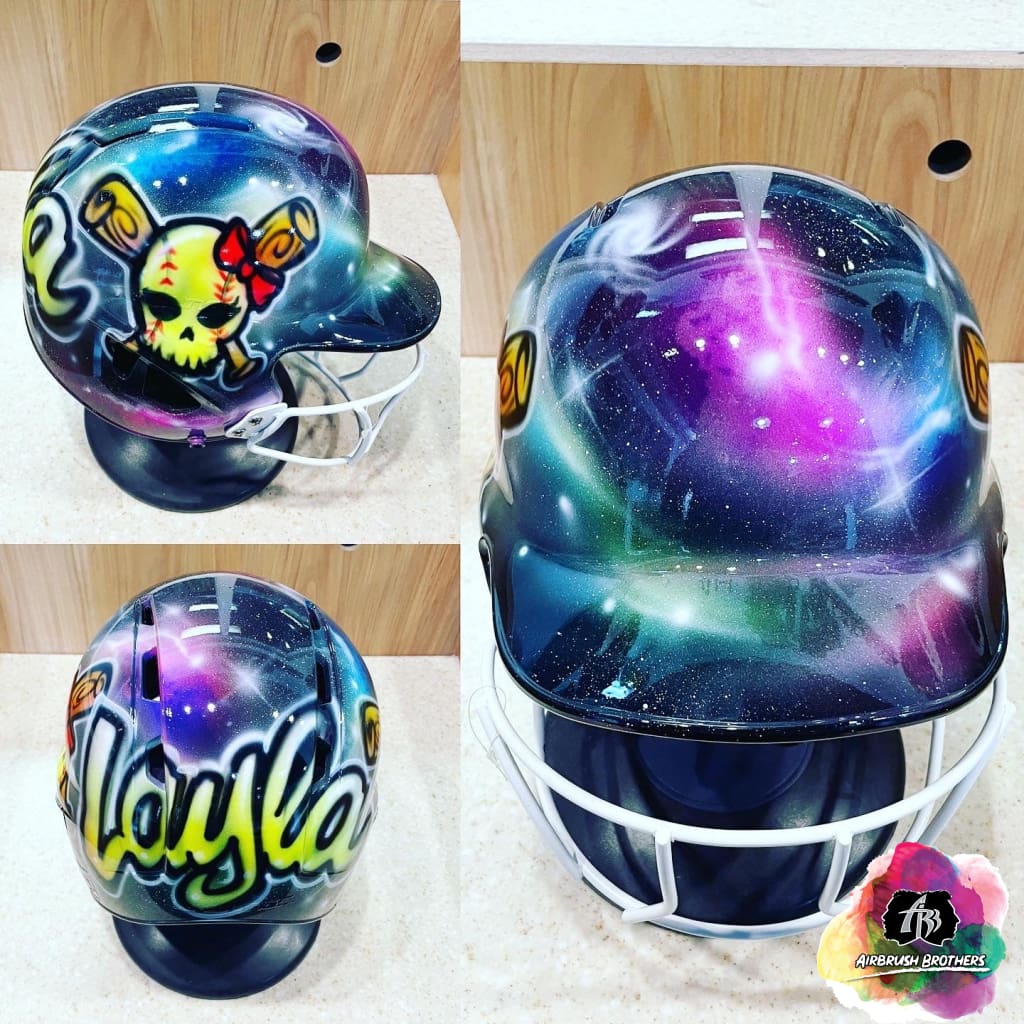The image showcases three views of a vibrant, custom-painted baseball or softball helmet resting on a stand against a wooden background. The helmet features a striking galaxy-themed airbrush design with an array of vivid colors, including pink, green, purple, and black. The front displays a white face guard, emphasizing the helmet's intended use in sports. Prominently, the helmet includes a personalized name "Layla" in bold, stylized yellow lettering across the back.

Each side of the helmet is adorned with a unique graphic of a softball turned into a skull, highlighted by red stitching that mimics that of a baseball. This skull graphic is accompanied by a red bow and baseball bats forming a crossbones design. The artistic design implies the helmet's use in baseball or softball, catering to someone named Layla. 

Additional details include the logo and name "Airbrush Brothers" at the bottom right corner of the image, along with their distinctive "AB" logo marked with paint splatters, suggesting that this custom helmet is part of their promotional work.